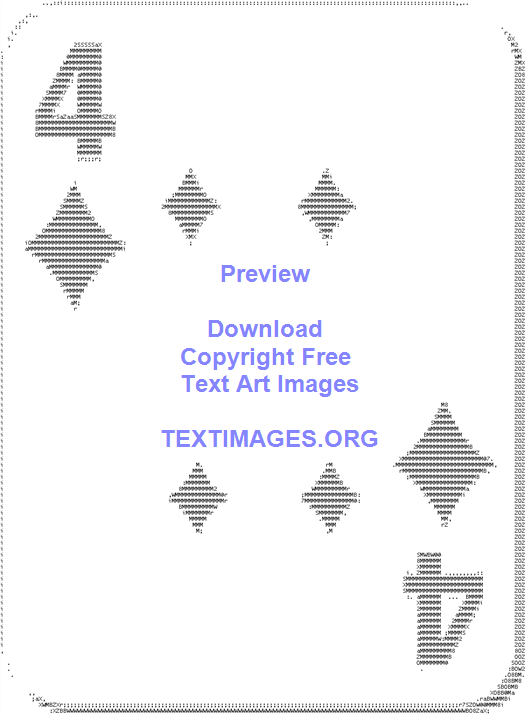This photograph features a digitally rendered black-and-white image of a four of diamonds playing card, reminiscent of old-fashioned ASCII art using zeros and X's. The card itself fills the entire frame and displays six diamond symbols arranged in the typical layout for a four of diamonds card. No real-world objects or people are present in the image; everything is computer-generated. Dominating the center of the image is a watermark that reads, "preview download copyright-free text art images textimages.org," suggesting that this image is an advertisement for the website textimages.org. The monochromatic design and the use of keyboard characters give the image a nostalgic, retro digital aesthetic.